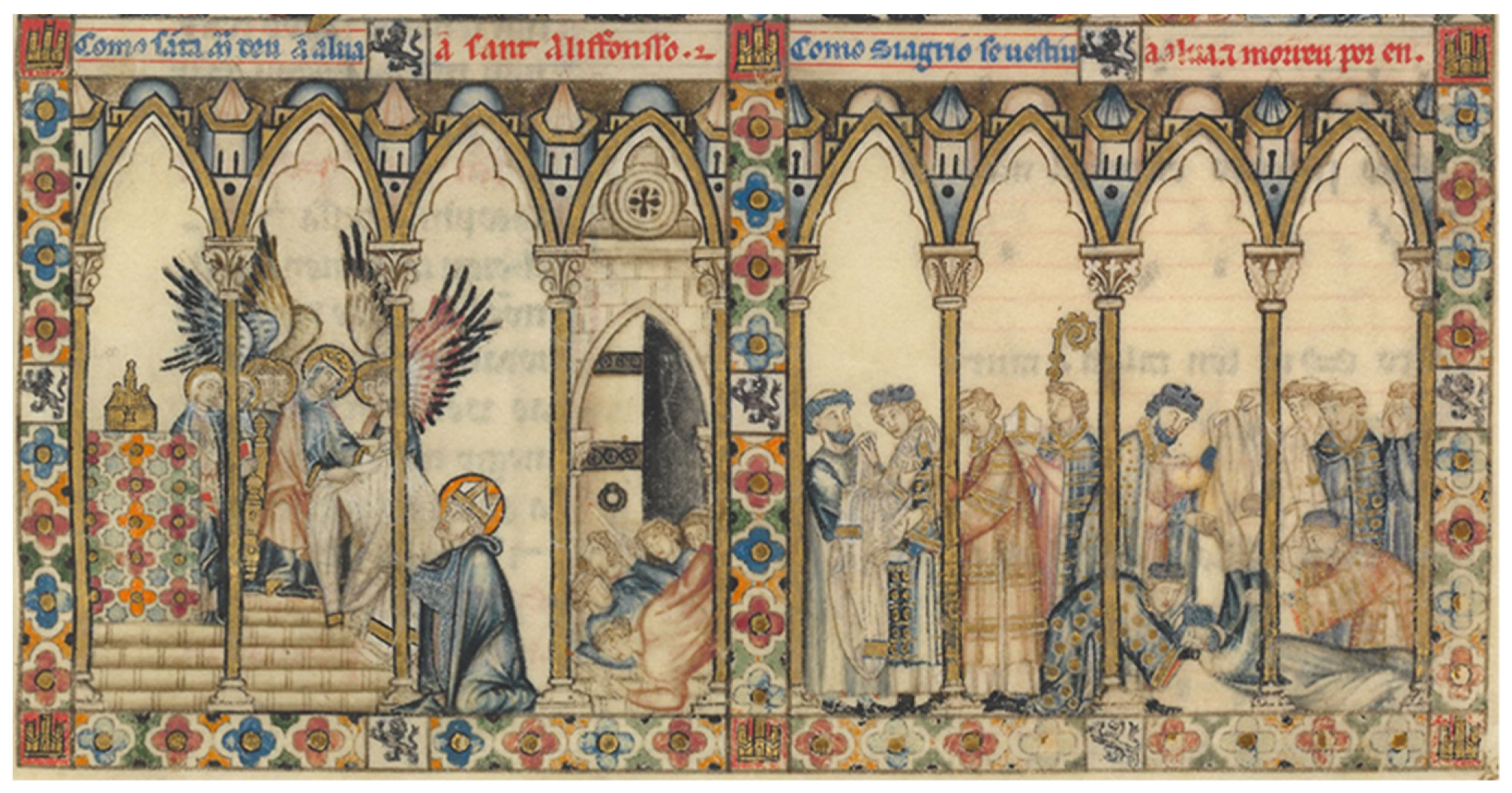This detailed medieval-style artwork, rich in historical and religious significance, features an elaborate and vibrant depiction of a religious scene. Emerging from a delicate, cream-colored or light tan background with multi-colored trims in blue, orange, and yellow, the image is divided centrally into two distinct sides, separated by a series of archways. At the top of the scene, intricate Latin manuscript handwriting, executed in a calligraphy style, seems to title or describe the events below.

On the left, an altar stands adorned with angels, their ethereal presence highlighted by halos above their heads. Kneeling at the altar, a man, possibly a king or a monk, gazes up in a state of prayer or supplication, his robes rendered in blues, whites, and reds.

The right side portrays a gathering of monks, priests, and possibly a figure carrying a Pope's hat and staff, engaged in what appears to be a solemn activity. They surround and tend to a person lying on the ground, seemingly ensuring their care or comforting them after a fall. This side of the image exudes a sense of communal concern and reverence.

The entire scene is encased in a floral frame, characteristic of the early medieval period, reminiscent of a precious page from an illuminated religious manuscript or a sacred text. The artist's use of various colors lends a dynamic quality to the depiction, enhancing both its aesthetic appeal and its historical authenticity.